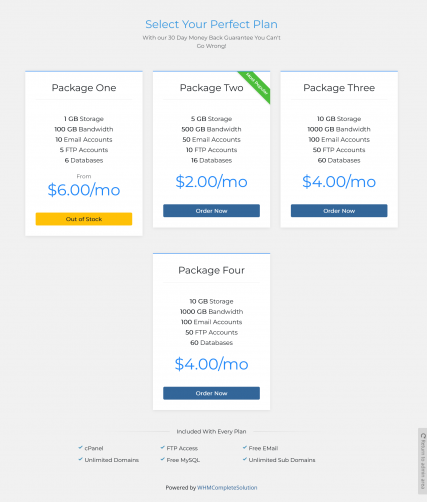The image displays a screenshot featuring a gray background with a prominent header that reads "Select Your Perfect Plan." Below this header, four different package options are outlined. The packages are organized in a 3x1 grid format, with three packages on the top row and one package on the bottom row.

- **Package One**: Listed at the top left, it includes 1 GB of storage, 100 GB of bandwidth, 10 email accounts, 5 FTP accounts, and 6 databases. The price is prominently displayed as "$6/month". Additionally, a yellow notification box at the bottom of this package indicates that it is "Out of Stock".
  
- **Package Two**: Positioned in the top center, this package is marked as the "Most Popular" with a banner on the right side. It offers 5 GB of storage, 500 GB of bandwidth, 50 email accounts, 10 FTP accounts, and 16 databases. Notably, it is priced at an economical rate of "$2/month".

- **Package Three**: Situated at the top right, this package costs "$4/month" and includes various features, which are not specified in the description but are different from package four.

- **Package Four**: Located on the bottom row, this package also costs "$4/month" and comes with its unique set of unspecified features distinct from package three.

The clear layout and concise information aim to help users compare and select the plan that best fits their needs.